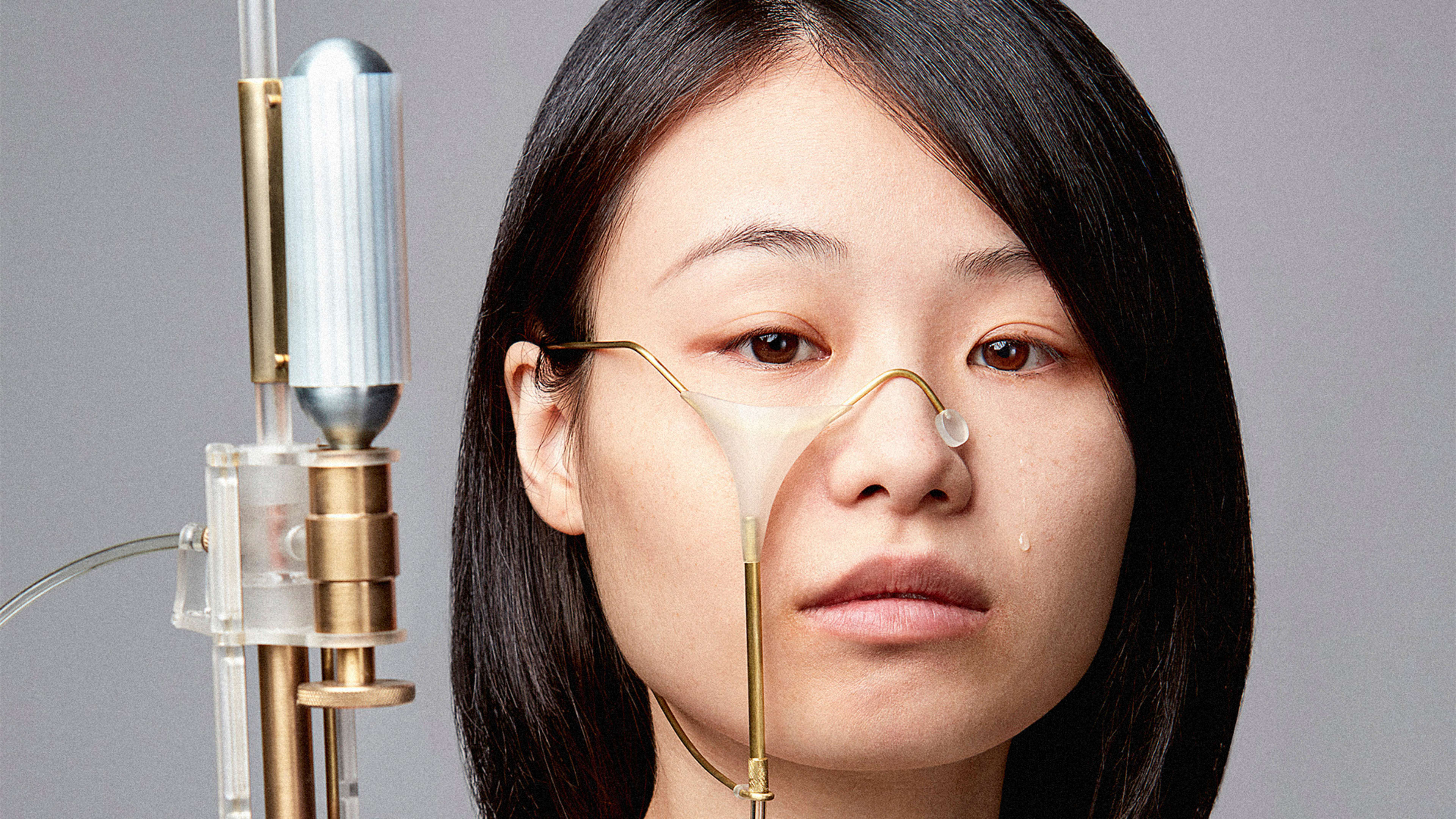The close-up, professionally lit photo depicts an upset and sad Asian woman with black-brown, straight hair and tan skin, showing only her head. A single tear rolls down from her left eye. She is surrounded by a complex, gold and silver medical-like device, contrasting beautifully with her brown eyes and the gray background. The device features a golden contraption with a white tip that arches over the bridge of her nose, partially attaching around her ear, without directly connecting to her nose or mouth. This apparatus is linked to a nearby cylinder and brass parts, through a series of tubes and knobs, implying a healthcare-related purpose. The lighting highlights every detail, although the exact function of the device remains ambiguous.